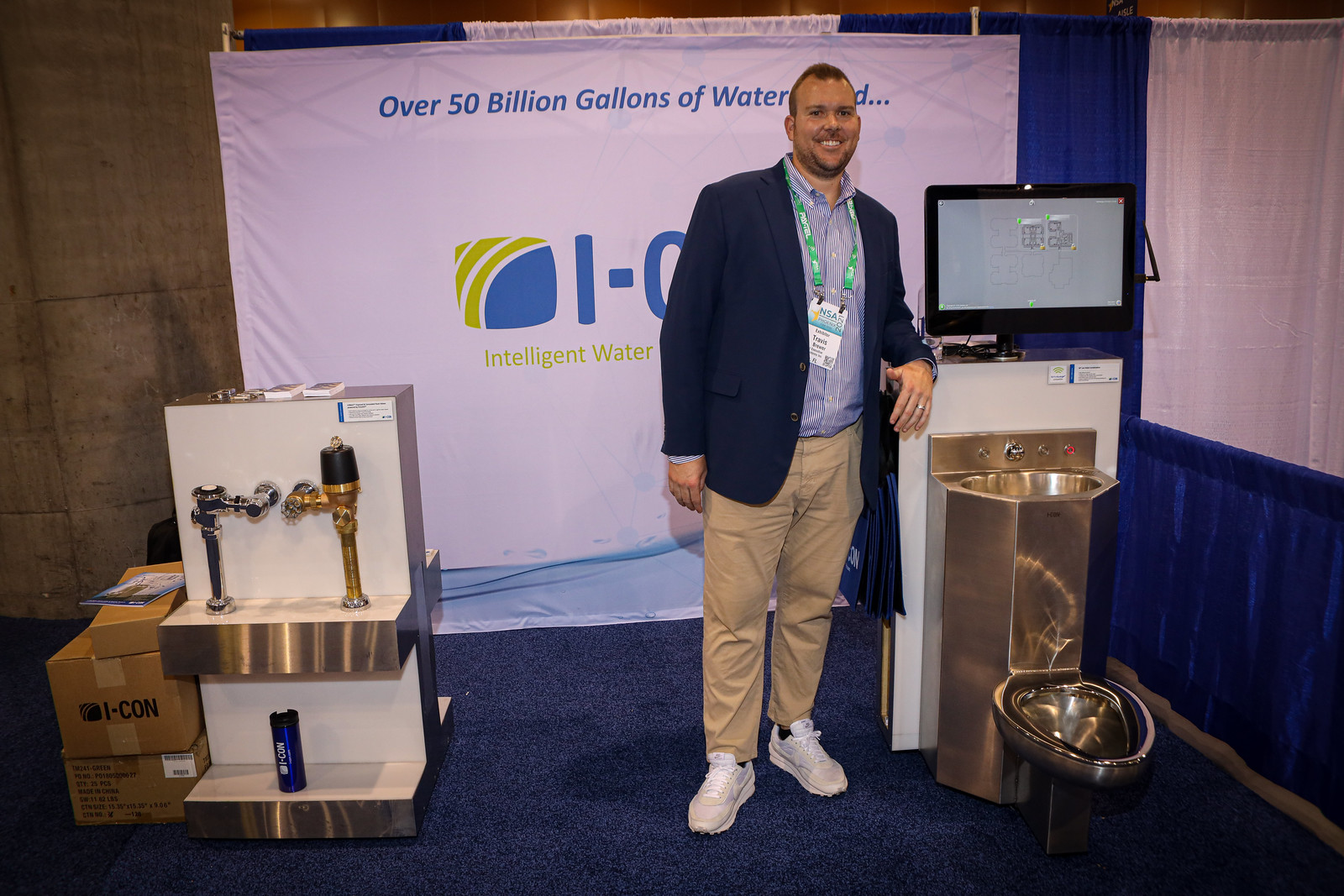The photograph features a smiling young man with fair skin, standing indoors on a floor covered with a blue carpet. He is dressed in a blue and white striped shirt, a dark blue coat, cream-colored pants, and white shoes. The man is positioned to the left side of a unique water fixture that combines a metallic golden sink and commode, which glistens with a shiny brown hue. His right hand rests on a table that supports a display monitor perched above the commode, further highlighting this innovative contraption. Behind him, a partially obscured banner reads, "Over 50 billion gallons of water... Intelligent Water," likely indicative of the company's focus on water-saving innovations. To his left, various plumbing fixtures, including golden and silver flushers, are displayed on an outcropped piece of metal, while some brown boxes are stacked nearby. This scene appears to capture an exhibition at a plumbing convention, where the man, possibly an exhibition promoter, showcases advanced bathroom equipment.